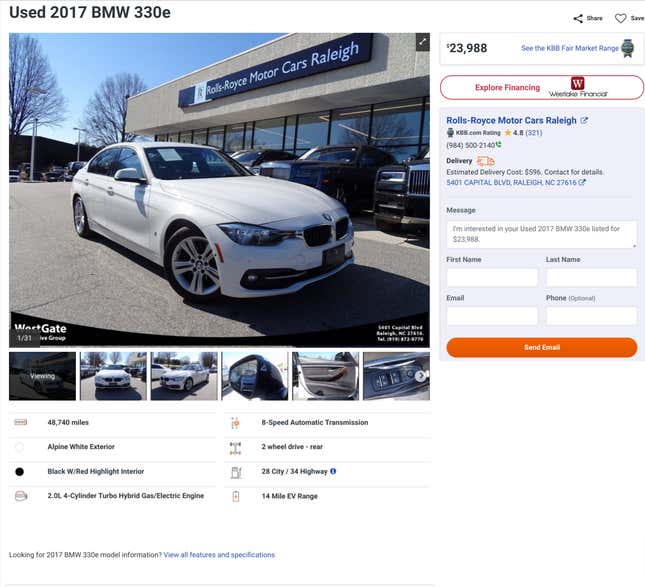Screenshot of a used car listing on Kelley Blue Book (KBB) website for a 2017 BMW 330e

In this detailed screenshot from the Kelley Blue Book (KBB) website, a listing for a used 2017 BMW 330e is prominently featured. The headline, set against a clean white background, reads "Used 2017 BMW 330e" with the "e" in lowercase. Below the headline, a primary image showcases a sleek, white BMW parked in front of a dealership. The car, which blends the aesthetics of a sporty vehicle with the practicality of a sedan, is positioned in front of a building marked by a gray concrete slab sitting above large glass windows and doors.

The dealership is identified by a blue sign with white lettering that reads "Rolls Royce Motor Cars Raleigh." Further down the listing, several smaller images of the car are displayed, including front and side views, as well as interior shots, providing a comprehensive look at the vehicle.

On the right side of the listing, the price of the car is prominently displayed as "$23,988." Adjacent to this price, in a light blue font, is an invitation to "See the KBB Fair Market Range." Beneath this section, the dealership name appears again: "Rolls Royce Motor Cars Raleigh." The estimated delivery cost is listed as "$596," followed by a prompt to "Contact for details."

Further down, there is an interactive section allowing potential buyers to send a message. The pre-filled text box reads, "I'm interested in your used 2017 BMW 330e, listed for $23,988." Below this, fields are available for the user's first name, last name, email, and an optional phone number. To finalize the message, an orange rectangular button with rounded corners at the bottom of the section reads "Send Email" in white text.